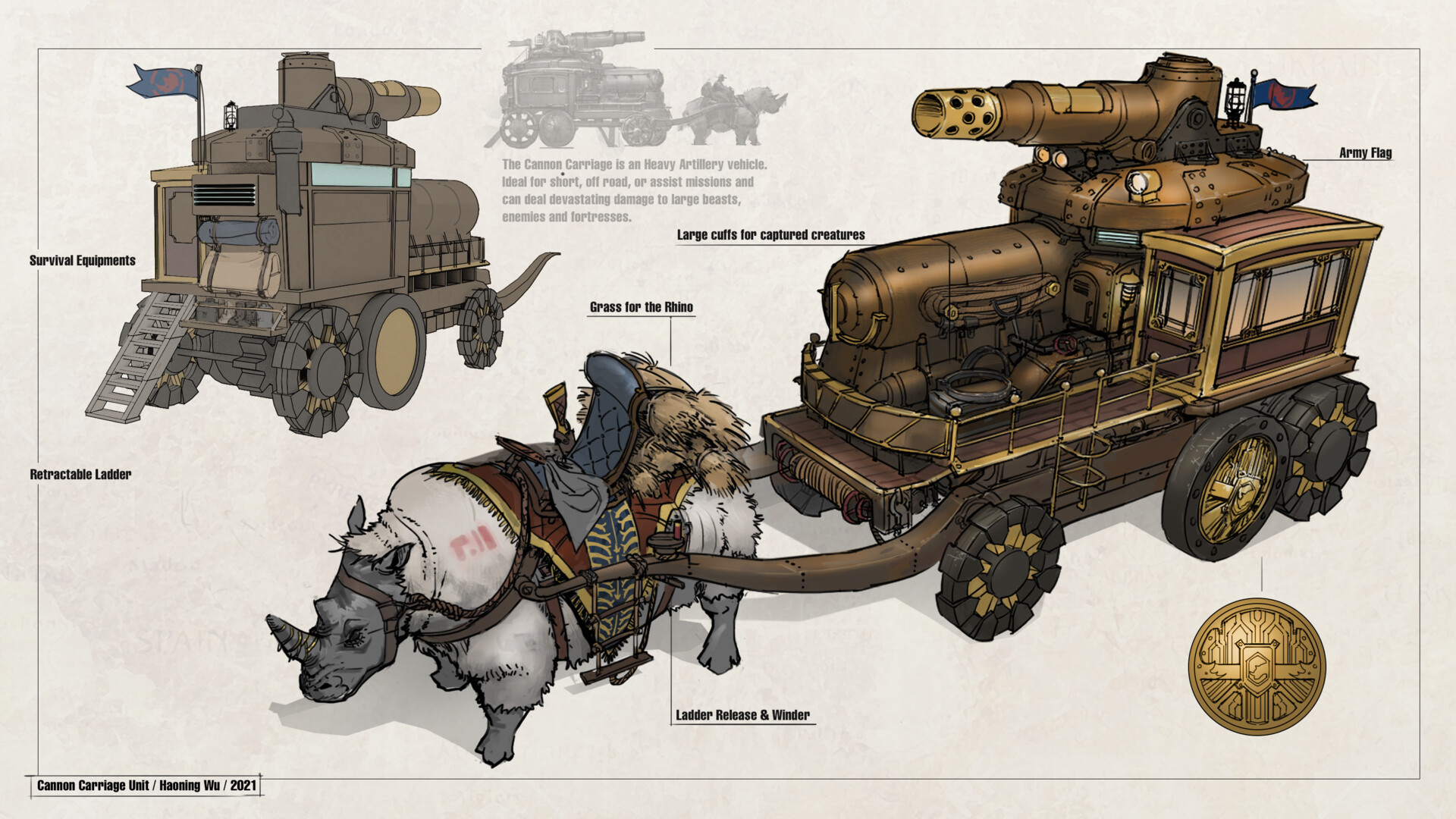The hand-drawn image, resembling concept art for a cartoon or video game, portrays a detailed steampunk scene with a wooly rhinoceros pulling a brass and bronze tank. The heavily adorned tank features large blocky wheels, a steam engine despite being rhino-drawn, headlights, a turret, and a small window. The tank's intricate design includes a section labeled "survival equipment," a back-side ladder, and a blue flag with a red design. The wooly rhinoceros, fitted with a blue stitched saddle and bundles of twigs or fur, pulls the tank while a brown rug and black leather seat rest on its back. The tan-beige background of the rectangular diagram is bordered by a thin black line, with numerous small, hard-to-read labels detailing parts like an army flag, ladder release and winder, and grass for the rhino. The annotated blueprint, rich with steampunk elements and unique flair, suggests a multi-functional vehicle with living quarters and a place for captured creatures. At the bottom of the page, the label reads "cannon carriage unit 2021."